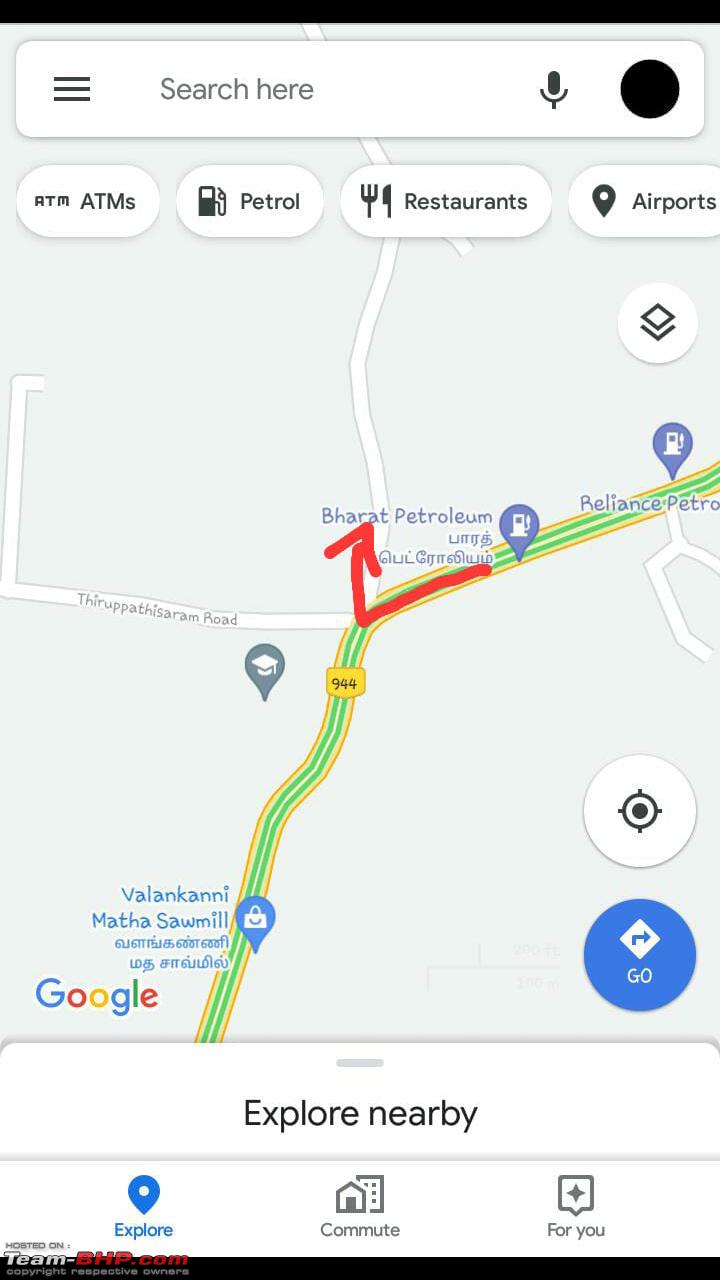This image is a detailed screenshot from a map application, possibly Google Maps, displayed on a mobile phone. The screenshot is in a vertical rectangular format, typical of a smartphone screen. 

At the top of the image, there is a white search bar. On the left side of this bar, there are three horizontal lines, followed by the text "Search here," a microphone icon, and a black circle. Below the search bar, there is a row of white buttons with black text, each representing different categories of local amenities. The first button displays "ATM, ATMs." The next button features a gas pump icon and the text "Petrol." The third button shows a fork and knife symbol with the label "Restaurants." The fourth button has a pin icon labeled "Airports."

The primary portion of the image is occupied by a map. The map depicts a major highway marked by green and yellow lines, identified as Highway 944. Various smaller roads intersect with the highway. Iconic markers are scattered across the map, notably on the right side. One gas station is labeled "Reliance Petro," and further down the road, another is marked "Barat Petroleum," with some supporting text not in English.

There is a road titled "Thirupastisram Road," along with the names of other locations, such as "Valankani Mathasawmill." 

Near the bottom of the image, nestled within the map, is the recognizable Google logo. Adjacent to it on the right side is a reticle icon, resembling a crosshair, likely used for centering the map. Below this is a prominent blue "Go" button. Further down, three more buttons labeled "Explore," "Commute," and "For You" are visible, providing additional navigation options for the user.

This detailed screenshot captures the essential features and functionality of a mobile mapping application interface.